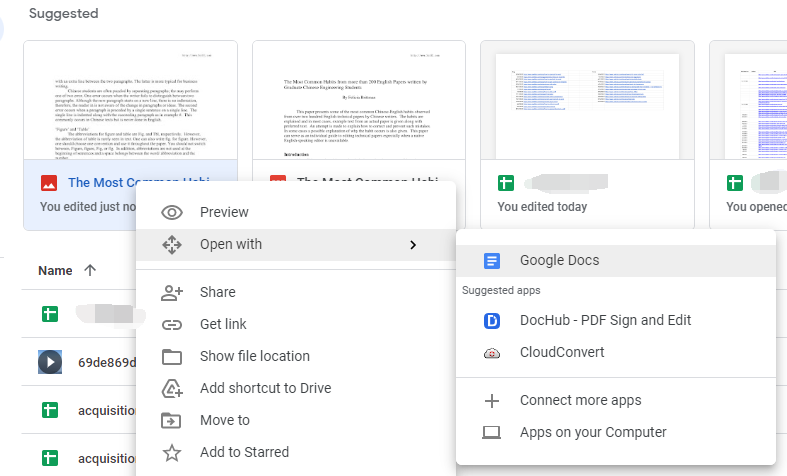A screenshot of a Google Drive interface, likely from a student's account, reveals several essays open in the background saved as Pages documents within Google Drive. The visible essay is titled "The Most C..." with the rest of the title truncated. The option to open this document with Google Docs is displayed, along with suggestions for alternative applications from Document Hub. An option to convert the document to another format using Cloud Convert is also present. Additionally, the interface shows multiple files recently added to the user's Google Drive, marked with green icons. The Drive features options for inserting numbers and images into the documents.